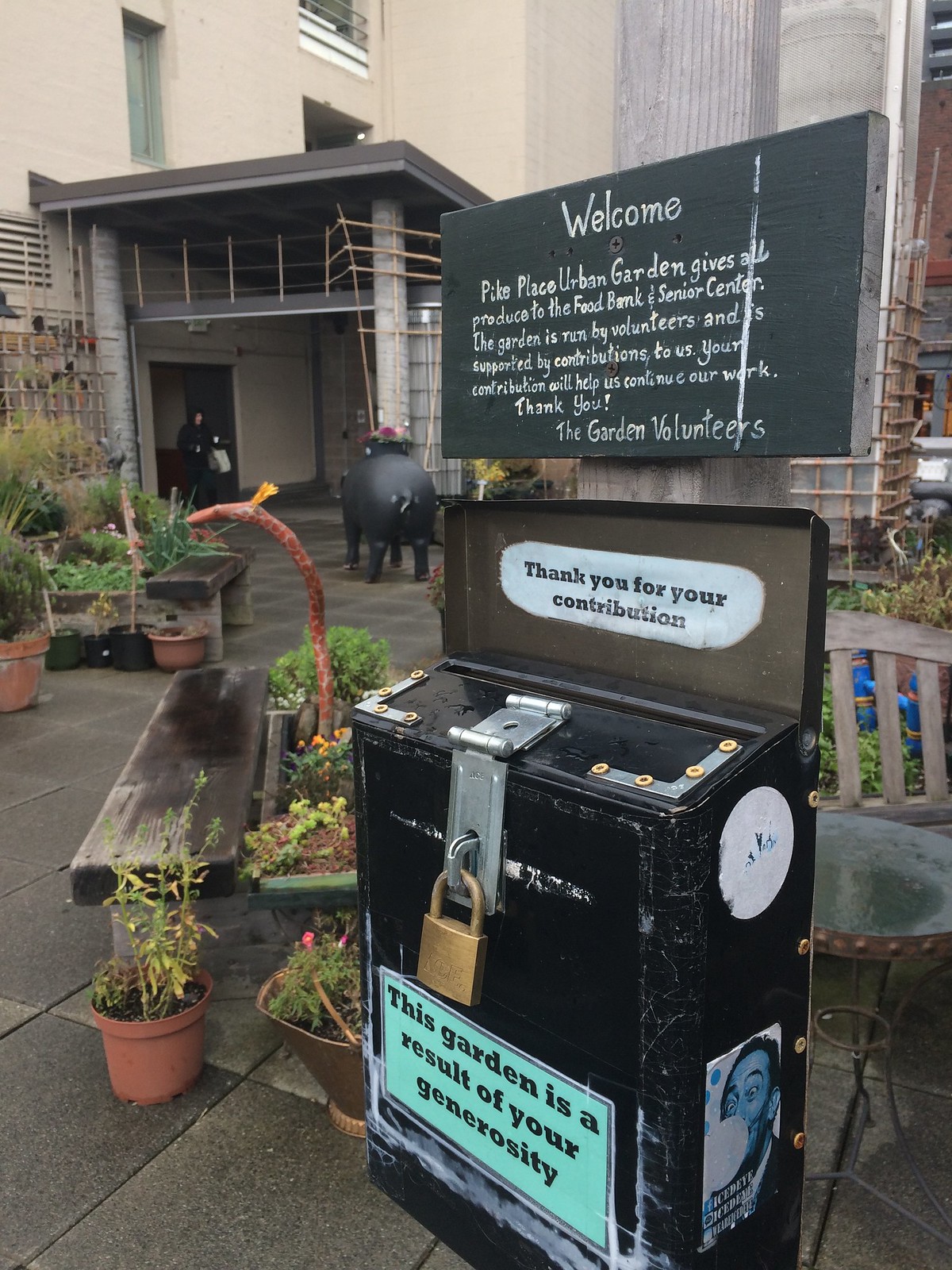The image depicts a tall, rectangular outdoor sign at Pike Place Urban Garden, mounted on a tall, gray wooden pole on the top right corner. The sign is black with white lettering that reads: "Welcome. Pike Place Urban Garden gives all produce to the food bank and senior center. The garden is run by volunteers and is supported by contributions to us. Your contribution will help us continue our work. Thank you, the garden volunteers." Below the sign, there's a large black donation box with an open lid that also reads "Thank you for your contribution." The box is secured with a brass padlock, and a green sign on the box states, "This garden is a result of your generosity."

In the background, there are several green potted plants and benches scattered around. A wooden bench-style table with additional potted plants on it is visible, along with plant boxes and a larger building in the distance. The outdoor setting features pavers on the ground, creating a welcoming environment enhanced by the garden's lush greenery and community-focused message.